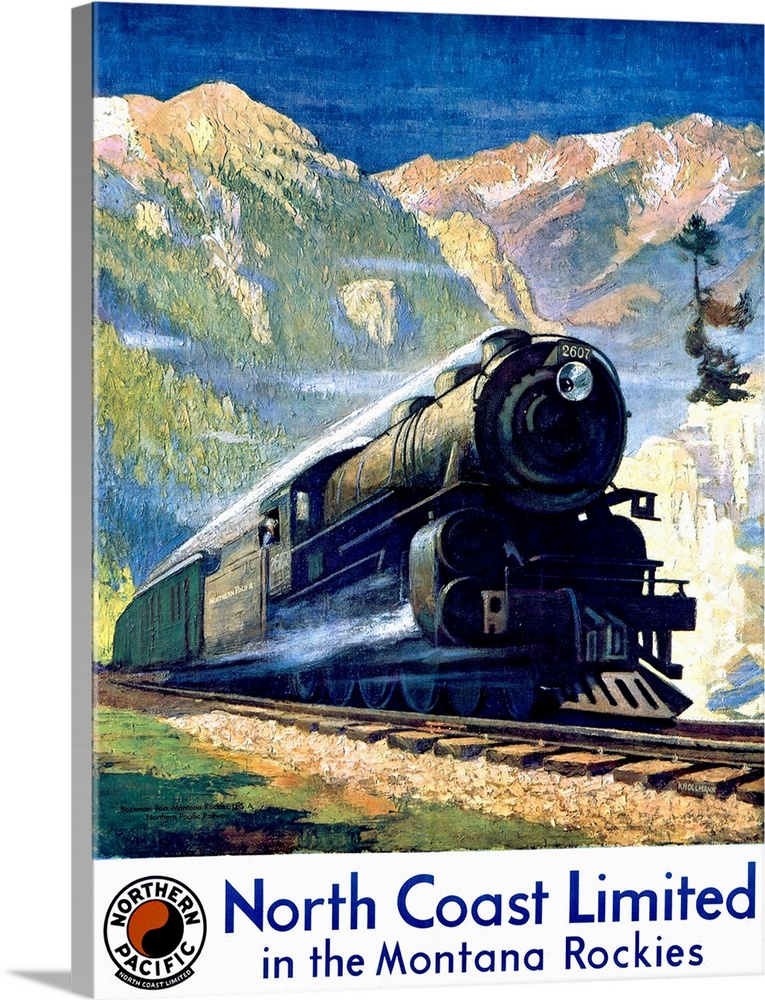The image appears to be an advertisement or the cover of a pamphlet for the North Coast Limited in the Montana Rockies by Northern Pacific. The central focus of the painting is an old-style steam engine, numbered 2607, barreling towards the viewer with noticeable speed. The engine, painted in black, features a barrel-like canister at the front and chimneys emitting visible steam. Trailing behind are green passenger cars. The scene is framed with a mixture of green, blue, and pink mountains in the background, accented with snowy peaks and trees, though the backdrop lacks fine detail. The railroad tracks are gray with brown wooden boards underneath. At the bottom, a round logo displays the Northern Pacific name and features a yin-yang symbol in the center. The text box prominently reads "North Coast Limited in the Montana Rockies," indicating the train line being showcased.